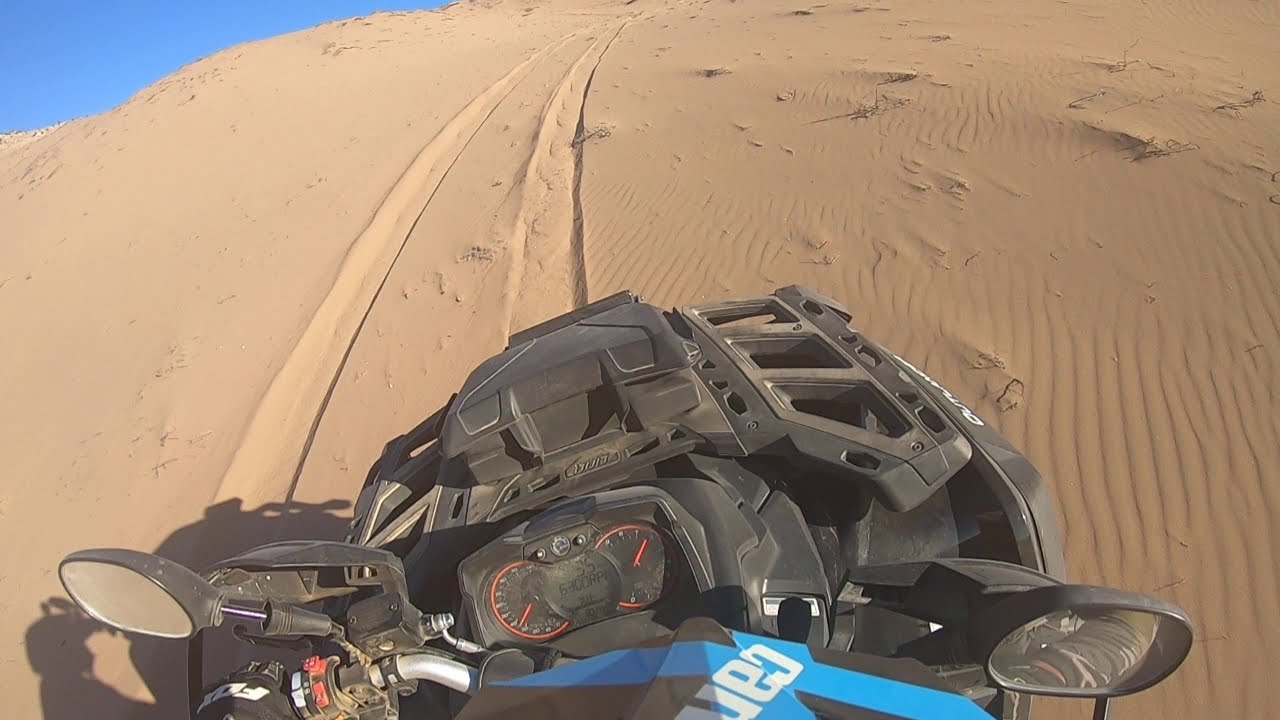The image captures a rider's perspective from an outdoor utility vehicle, such as a four-wheeler or an all-terrain vehicle, navigating through a sandy desert landscape on a bright, sunny day. The partial view of the vehicle reveals numerous gray metal parts at the front, including handlebars, rearview mirrors on either side, and a speedometer. The left hand of the rider, gloved, grips one of the handlebars. White text on the vehicle reads "C-A-N," and a blue marking is also visible. The sandy terrain ahead, showing windblown patterns and traces of narrow tracks, unfolds towards a tan brown sand dune with sparse, straggly grass. The rider's shadow, donning a helmet with a mounted camera, is cast on the sand below. A vivid, deep blue sky occupies the upper left corner of the image, creating a striking contrast with the desert's golden hues.